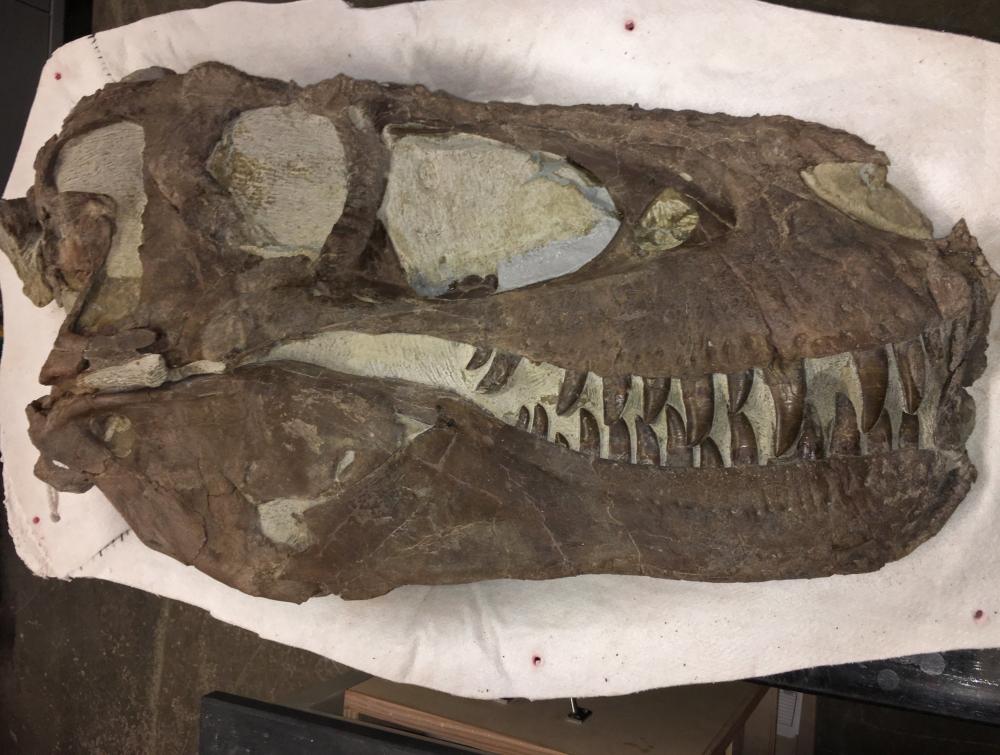The image depicts a fossilized dinosaur skull, likely belonging to a T-Rex, positioned centrally on a table within an indoor setting. The skull, primarily dark brown with patches of grayish white and light brown, features several sharp teeth, though some are missing. Notable are the several holes where eyes and other structures once were, giving the skull a distinct, aged appearance. Its mouth is closed and it faces the left side of the picture. The table beneath the skull is covered with a white linen cloth, irregularly shaped, with hints of wood peeking through and perhaps a small switch visible. The overall scene appears to be staged, possibly for an exhibit or display in a museum.